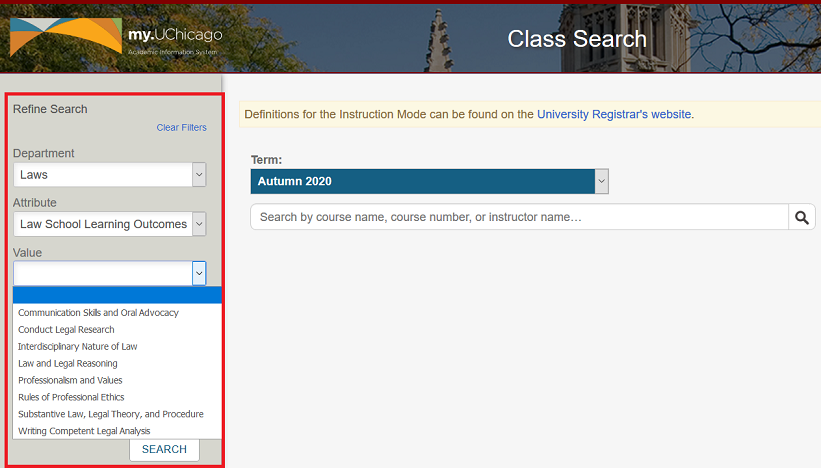This landscape mode screenshot, likely taken from a laptop, captures a webpage from the My.UChicago site. Dominating the upper section is a vivid, professional photograph of an outdoor autumn scene. The image features a tree with vibrant orange leaves on the left and a partially bare tree with a few green leaves on the right. Centered in the background, a building with a steeple adds an architectural element, while a stone cupola building is also visible on the right. Overlaid on this scenic header, in white text, are the words "Class Search," and the My.UChicago logo is situated in the upper-left corner, though the text beneath the logo is not legible. This entire top portion is underscored by a prominent red stripe.

Beneath this image, the webpage is divided into two main columns. The left column has a dark gray background and features a red-highlighted section. This section includes options to refine the search, with selections such as "Department" with "Laws" chosen, and "Attribute" with "Law School Learning Outcomes" selected. It also offers a menu to choose values like "Communication Skills," "Conduct Legal Research," "Interdisciplinary Law," "Professionalism Rules," "Substantial Law," and "Writing Competent," along with a blue search button at the bottom-right of this highlighted area.

The right column sports a lighter gray background and includes a section labeled "Definitions for the Instruction Book" with a live light blue link to the "University's Registered Website." Below that, a green-background box specifies "Autumn 2020" as the term. A search bar underneath invites users to "Search by course name, number, or instructor's name."